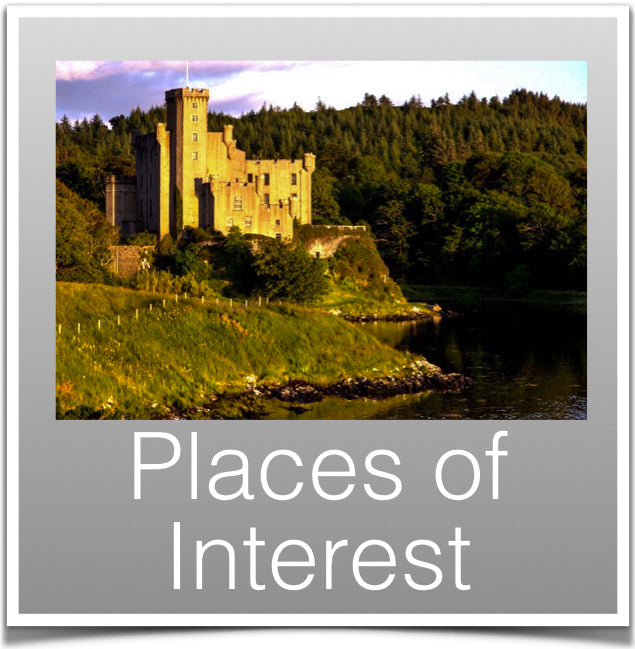In the photographic image, we observe a picturesque castle, likely situated somewhere in the British Isles such as Scotland or Ireland. The setting appears to be late afternoon or possibly during sunrise or sunset, adding a unique warm glow to the landscape. The castle, modest yet stately, features a tall, square-shaped main tower with four sets of windows and what looks like a post at the very top. Accompanying the tower, there are other turrets, a brick wall, and a chimney, all contributing to its historical appearance.

Nestled on a bluff, the castle commands a view over a dark body of water, adding a serene yet dramatic element to the scene. In the background, lush, green trees form a dense forest beginning to show hints of fall. The sky above reflects a striking contrast, with the left side painted in deep blue hues while the right side transitions to a white, cloudy atmosphere. 

The structure itself is perched atop a hill, with what may be white stakes or fences lining the path leading up to it. The castle's yellowish façade catches the sunlight, enhancing its regal and ancient charm. Framing the image, a grey border with a white outline at the bottom contains the text "Places of Interest" in white letters. This caption blends seamlessly with the overall tranquil yet majestic ambiance of the photograph.